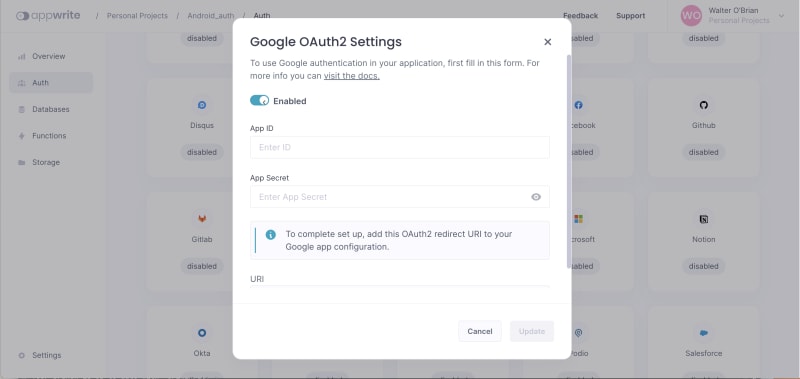This is a detailed descriptive caption for the image:

The image displays a settings page of an application project, specifically focused on Google OAuth 2 settings. The background of the image is a primary settings page, slightly grayed out to highlight a smaller, more prominent settings box in the foreground. At the top of the background page, the navigation path reads "app / personal project / Android_auth / auth." A vertical navigation bar on the left features various sections including "Overview," "Auth," "Databases," "Functions," "Storage," and at the bottom, "Settings." Scattered in the background are several service integration options like Discus, Git, GitLab, Okta, Facebook, Microsoft, Salesforce, Notion, and GitHub.

In the foreground, the highlighted smaller box is titled "Google OAuth 2 Settings." The instructions within this box state: "To use Google authentication in your application, first fill in this form. For more info, you can visit the docs" with the "visit the docs" text underlined. The settings indicate Google OAuth 2 is enabled, shown by a toggle button. Below this, two labeled fields are provided: "App ID" with an entry box labeled "Enter ID," and "App Secret" with an entry box labeled "Enter app secret." Another note advises: "To complete setup, add the OAuth 2 redirect URL to your Google app configuration," with a space provided for entering the URL.

At the bottom of this smaller box, there are two buttons: "Cancel" and "Update," with the "Update" button currently grayed out, indicating it is not active or clickable at this point.